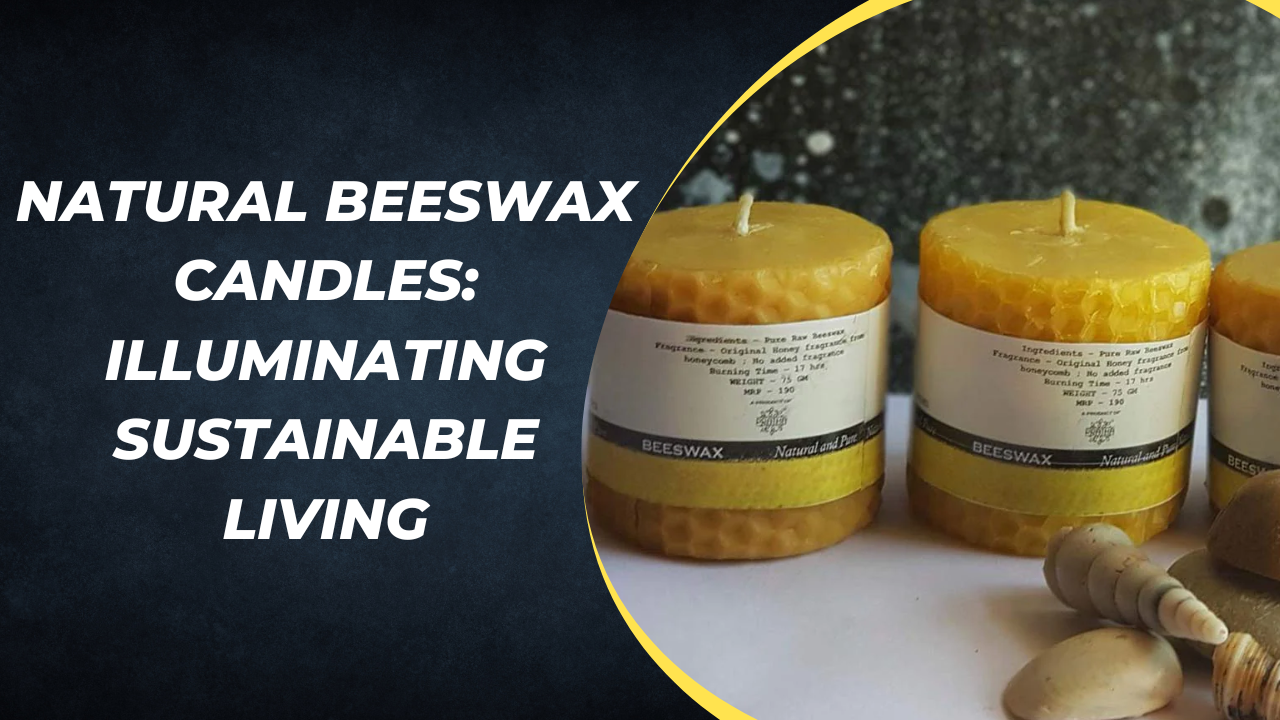The advertisement for natural beeswax candles features a sleek design with text to the left, which reads, "Natural Beeswax Candles Illuminating Sustainable Living." On the right, there are three light brown or yellow-brown beeswax candles, each with a white, black, and yellow label prominently displaying the word "beeswax." The candles are arranged on a white surface, surrounded by seashells, against a backdrop that transitions from gray at the bottom to blue midway, sloping upwards to the right. The wicks of the candles are unburned, enhancing their pristine appearance. The overall layout and aesthetic emphasize the sustainable and natural appeal of the beeswax candles.